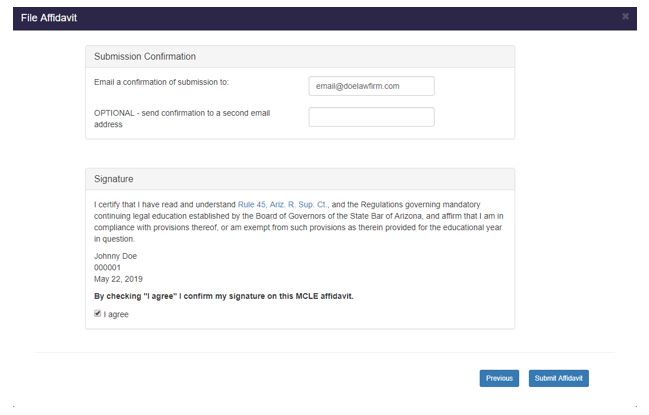In this image, we are looking at a detailed screenshot of a form interface titled "AFFIDAVIT." The title is prominently displayed in white text in the top left corner against a dark bluish background that spans the entire top section of the screen. On the top right corner, there's a small gray "X" icon.

Beneath the header, the form is divided into several sections. The first section is labeled "Submission Confirmation," followed by another section titled "Email Confirmation." In this section, there is a rectangular input field where one can enter an email address for submission confirmation. Directly below, there's a section for an optional second email confirmation, with another rectangular input field to the right.

The next section is the "Signature" area. It contains a detailed statement: "I certify that I've read and understand Rule 45 ARIZ R-S-U-P-C-T and the regulations governing mandatory continuing legal education established by the Board of Governors of the State Bar of Arizona and affirm that I am in compliance with provisions thereof or am exempt from such provisions as they're provided for the educational year in question." This statement is followed by a signature line marked as "Johnny Doe, 500001, May 22, 2019."

To confirm the signature, there is a checkbox labeled "I agree," which is already checked off, indicating that the user has agreed to the terms and conditions stated above.